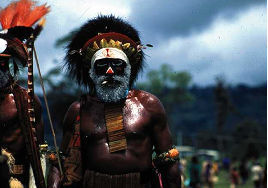The photograph captures a close-up image of a dark-skinned man, likely from an African or Aboriginal tribe, adorned in ceremonial attire. His face is prominently decorated with white face paint, outlining his eyes and nose, which also features a striking red trim. He sports a white, powdered beard that contrasts sharply with his skin. Atop his head, he wears a headdress composed of black fur adorned with burgundy ribbing and golden baubles. 

A beaded necklace cascades down the center of his chest, from just below his chin to above his belly button, and he has multicolored armbands near his elbows. He holds a bow in his right hand, although it lacks an accompanying arrow. Adding to his intricate ensemble, he has a strap that appears to be part of a bag draped over his right shoulder.

The background reveals a verdant landscape with blurry figures and trees, set against a skyline of blue sky interspersed with dark and white clouds, and possibly a distant mountain range or tall hills. Another individual in the background also wears white face paint and a headdress, underscoring the ceremonial nature of the scene.